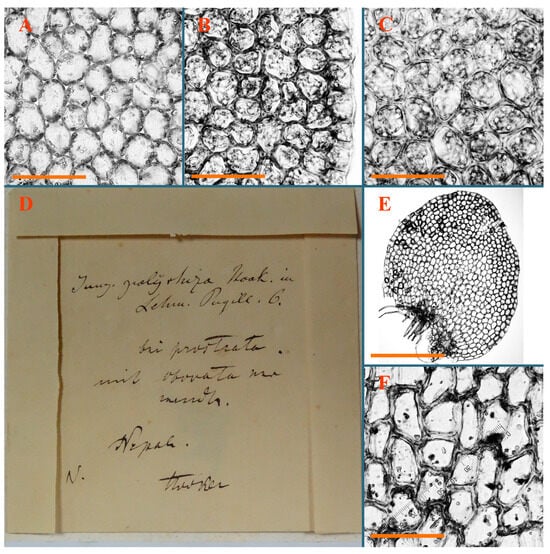This image presents a structured layout consisting of a series of labeled illustrations that potentially depict microscopic cellular structures in black and white, possibly as detailed drawings rather than photographs. Along the top row, there are three equally-sized squares labeled A, B, and C in red at the top left corners. Square A shows a close-up of white scales with gray divisions. Square B, similar in layout to A, appears sketchier and slightly darker. Square C, also resembling A, features more spread-out shapes with less defined lines between them. 

In the bottom row, there are two squares and a large square on the left. Square E, found directly below C, contains a depiction similar to A and C but appears more zoomed out, showing an array of small circles and shapes forming an oval border. Square F, to the right of E, resembles the box labeled B but with slightly larger, more zoomed-in shapes. To the left of E and F, the larger, four-square-sized box contains a piece of beige paper with black, cursive writing that is too small to be legible.

The overall arrangement suggests a methodical illustration of varying magnifications or conditions of similar cellular or molecular structures, important for scientific analysis or educational purposes. The writing on the larger beige paper appears to add a historical or explanatory context to the visual data presented in the smaller squares.